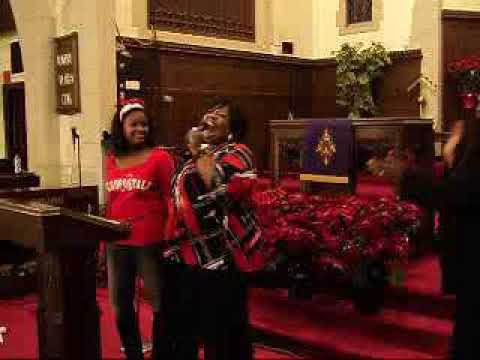The image depicts the interior of a church, featuring two Black women standing together, likely participating in a service. The woman on the left, who appears to be singing or speaking into a microphone held in her left hand, is wearing a festive red and black top, possibly adorned with a Christmas print. She also seems to be wearing a Santa hat or some form of headgear. The younger woman standing to her right has dark black hair and is dressed in a red and white top. The background shows light beige walls with brown furnishings, accompanied by a vibrant array of flowers and plants that add color to the scene. The floor is covered with a red carpet, and a brown podium stands in front of the women. The image's quality is somewhat low and pixelated, with the right side partially cut off, possibly showing another person. No text or numbers are visible.

In addition to this photo, the collection also includes a small square thumbnail icon indicating an image that has failed to load. This icon features a folded-over upper right edge, a white circle on a blue background in the upper left corner, something greenish in the lower left corner, and a white diagonal bar extending from the lower right corner to the middle right side of the image.